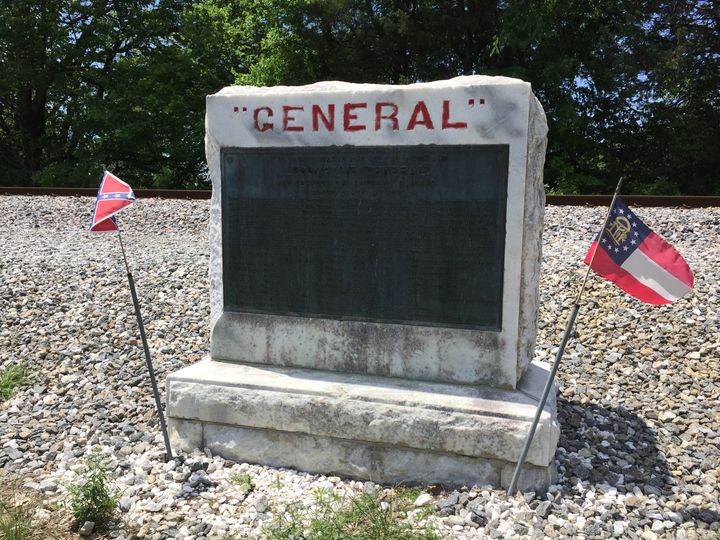The image depicts a standing headstone against a backdrop of trees and a blue sky, surrounded by small gravel pieces. The headstone, predominantly a whitish-gray color with dirt marks along its bottom, prominently features the word "GENERAL" in red, capital letters carved at the top. Below this, a large section of the headstone has an illegible text on a black background due to the poor lighting. Two small flags are placed on either side of the headstone, held up by metal stakes. The flag on the left resembles elements of the British flag with red diagonal lines on blue, while the flag on the right is a variant of the American flag, featuring alternating red and white stripes with a blue section displaying a building and stars. Small gravel pieces and higher terrain cover the foreground and background, with train tracks and trees lined up behind the grave site.